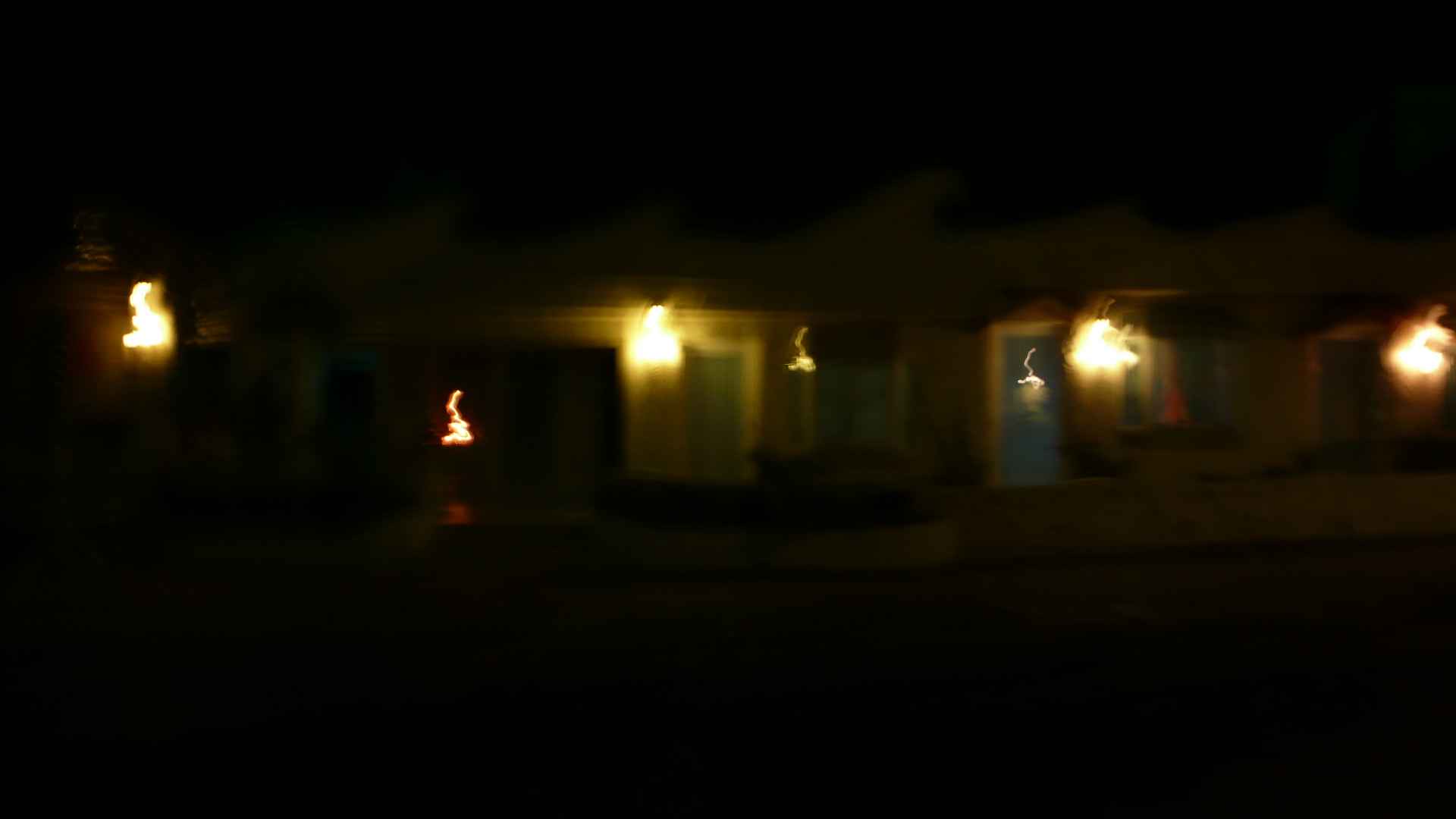The image is a blurry nighttime photograph of a row of adjoined houses or possibly a one-story motel. The sky is pitch black, and the ground below appears as a dark, almost blackish-gray surface, likely a mix of street and sidewalk. Each house features a front door, with the doors varying in shades of blue. Next to each door is a light fitting, each turned on, casting bright, random-shaped blobs of yellow light in the photograph. The roofline of the buildings is indistinct and seems wavy, possibly due to the blur. In front of the structures, there is a low-height wall with planters containing low bushes. The overall scene is dominated by the darkness, punctuated by the lights near the doors, creating an impression of quiet, nighttime ambiance.